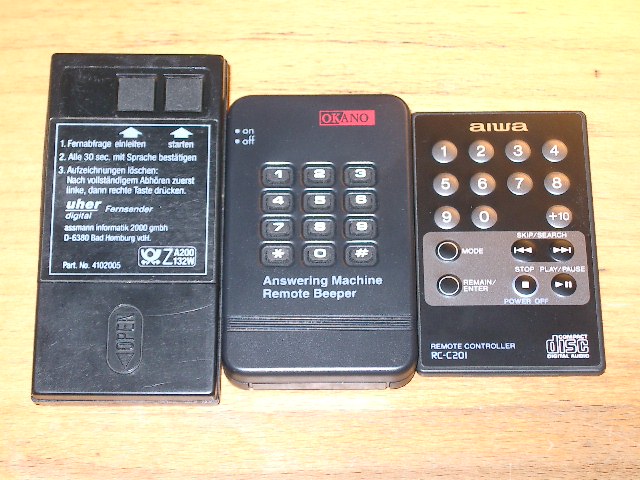The image features three vintage remote controls from the late 1980s or early 1970s, arranged in a row on a light-colored wooden surface. 

On the left is a black UHER remote, turned to showcase its back, displaying a white box with small white text. The text includes non-English language phrases and mentions "digital" and "multi-spec." 

In the center is an Okano remote, marked in black and red, noted for its functionality as an answering machine remote beeper. This remote features a numbered keypad (1-9, with 0), and designated buttons for on/off, pound, and star, along with text indicating it has a three-step process labeled one through three. 

The right-hand side hosts an AIWA remote control, primarily black with assorted buttons including mode, enter, skip, search, stop, play, and pause, specifically designed for a compact disc player. Below the array of buttons, it prominently displays the model RC-C201 and the words "remote controller."